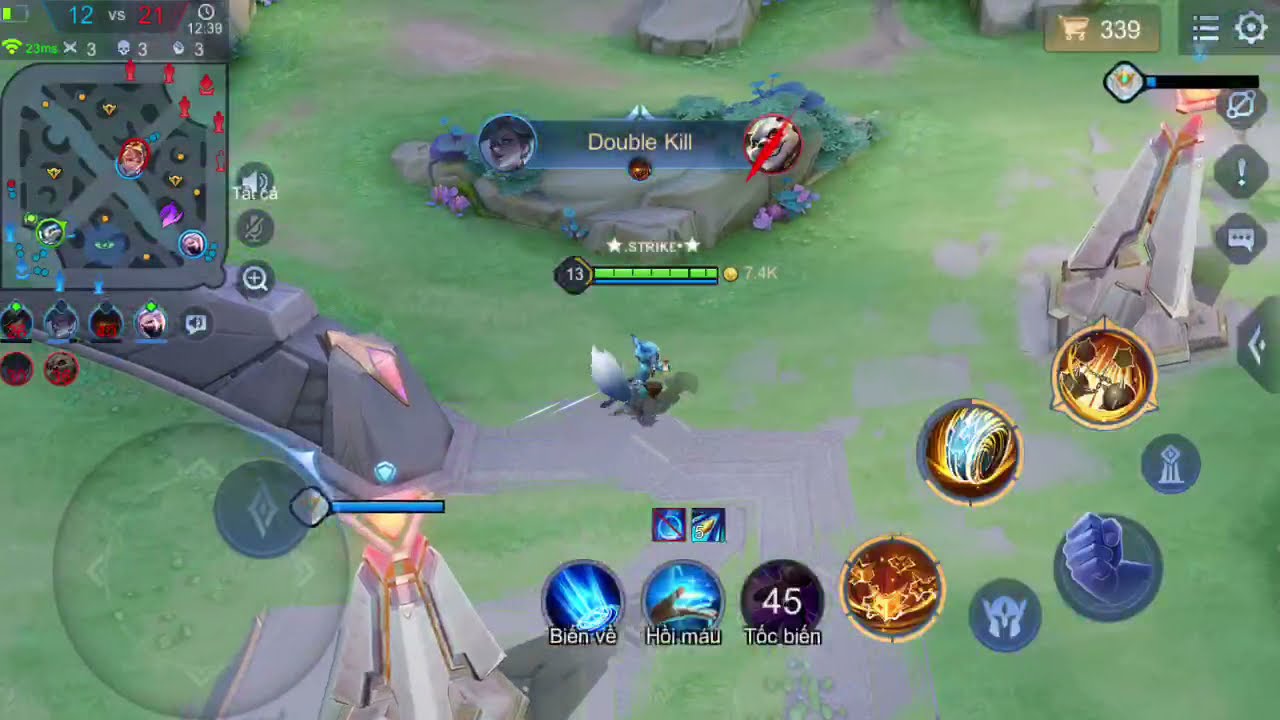This is a detailed screenshot of a video game in mid-play. Central to the image is a character resembling a fox with electric blue fur and a white tail, positioned against a green landscape dotted with gray rocks. The character is flanked by gun turrets that are gray with accents of gold, yellow, and pink. Above the character, there's a bar possibly indicating health or status, and the scene includes a rock formation directly above, another turret to the right, and a rock barrier to the left. 

In the top left corner of the screen, a section of the map is visible, displaying red and green markers that likely indicate object positions within the game. The text "double kill" is prominently displayed near the top center, highlighted by a power bar that mentions "strike," flanked by images of a young woman on the left and a dog resembling a pit bull or bulldog on the right. The power bar contains two stars and a pentagon with the number 13. 

At the bottom center and bottom right of the screen, there are various buttons and stickers with different emblems and writing, some of which appear to be in Vietnamese (phrases like "Bien Ve Ho Mau Tak Bien"). The icons are mostly round, featuring hues of blue, red, and orange, including graphics such as a fist and a tidal wave.